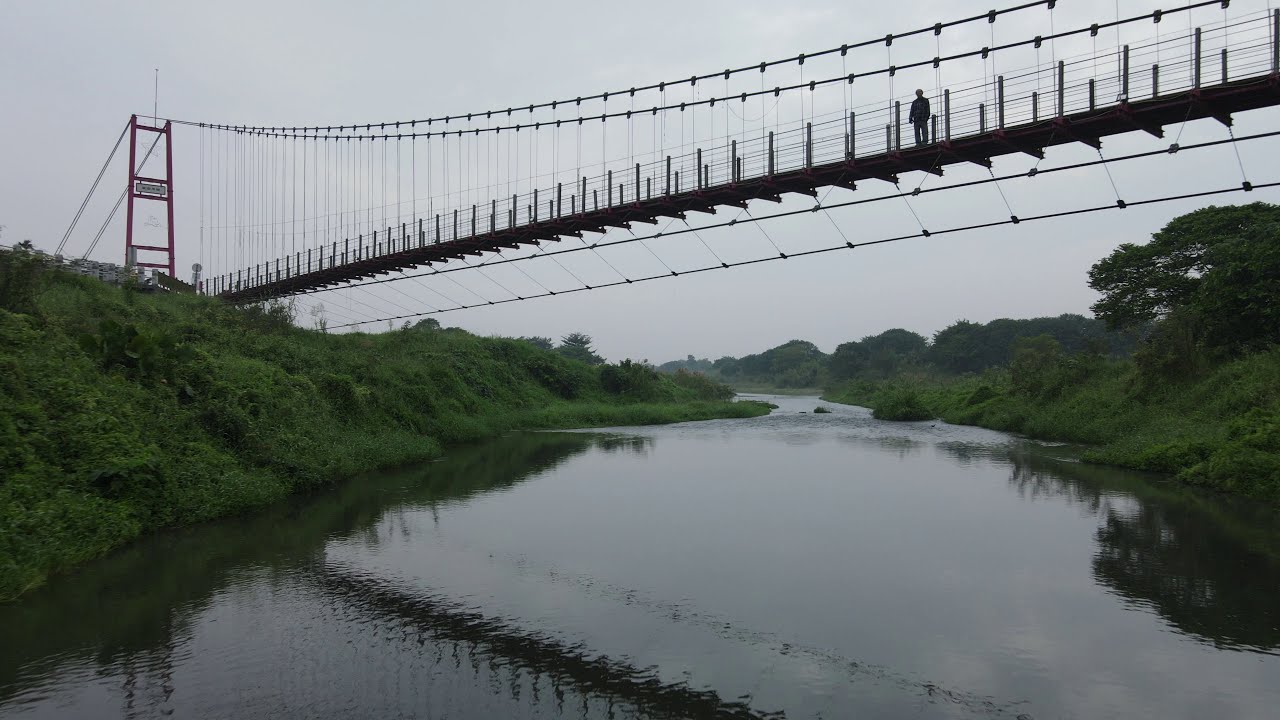The image captures a detailed scene of a suspension footbridge spanning over a gentle, slow-flowing river surrounded by lush greenery. Viewed from a low vantage point, likely on the side of a hill, the river extends into the distance, bordered by thick vines and various trees and shrubs that blanket the riverbanks. The bridge, featuring a distinctive suspension design with high, red support poles and numerous cables that slope gracefully in a concave pattern, reflects in the calm water below. The scene is set on an overcast day, casting a gray hue over the sky and emphasizing the vibrant green landscape. In the middle of the bridge stands a solitary person, seemingly looking in the direction of the camera, adding a focal point to the somber yet vividly green surroundings.